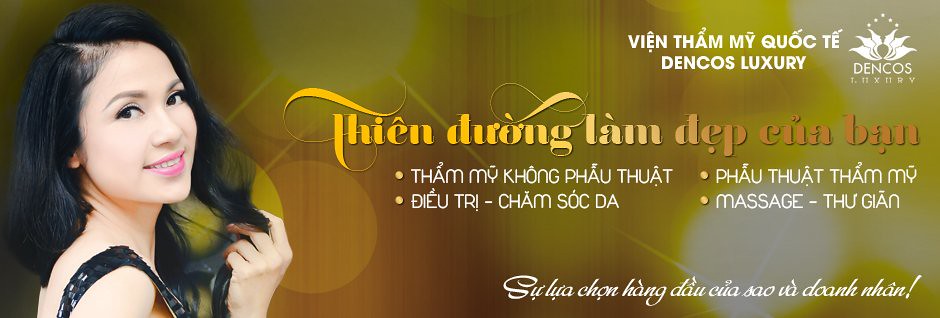The banner is a luxurious advertisement likely for a massage parlor or luxury service, characterized by a striking gradient of gold and yellow hues with darker gold transitioning into lighter yellow and back to darker gold. Intriguing light reflections or glares embellish the background, enhancing its opulent feel. On the left side, a woman with black hair, styled by twirling with her hand, poses gracefully in a thin-strapped black sequin dress and pink lipstick, her body angled to the right while gazing at the camera. The right side of the banner is filled with text in a South Asian language, and includes “massage” among other words. The top right corner features a stylized cartoon lotus flower with the phrase "Denko's luxury" prominently displayed underneath. The entire layout sprawls horizontally, underscoring its compelling promotional design.